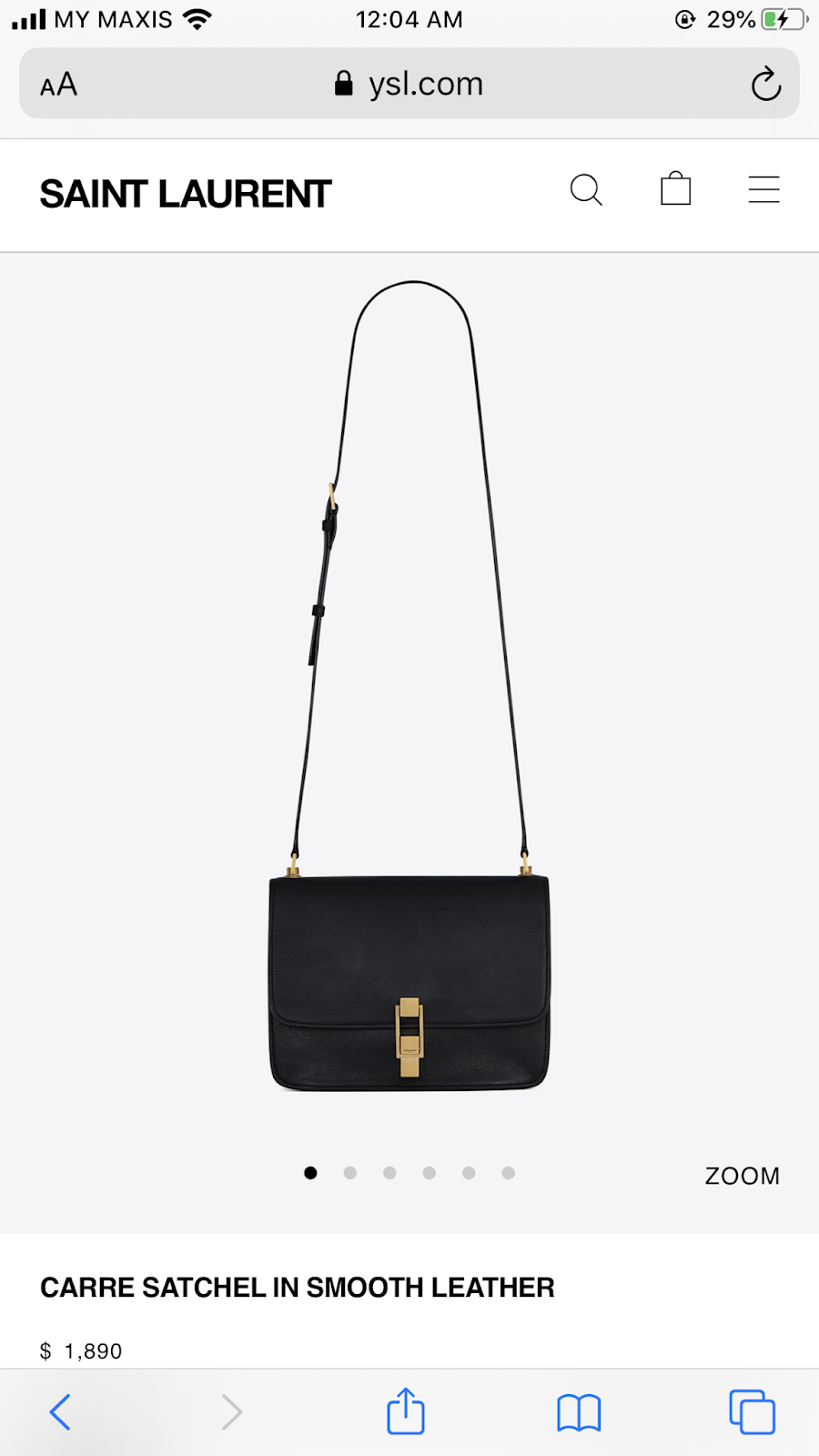The image displays the screen of someone's phone while browsing the Yves Saint Laurent website. The main focus of the image is a detailed photograph of a Yves Saint Laurent black over-the-shoulder bag. The bag, prominently featured, has gold buckles and a long strap, exuding elegance on a light gray backdrop. 

At the very top of the screen, the status bar reveals that the phone is connected to the Mi Maxis carrier, showing a strong signal with four bars and 4G connectivity. The time is precisely 12:04 a.m., and the battery indicator shows 29% remaining.

Just below the status bar, the user is on the Yves Saint Laurent official website, indicated by the URL "YSL for YvesSaintLaurent.com" displayed on a light gray background. To the left of the URL, there is an option to adjust the font size, and to the right, a refresh button. 

The main body of the image showcases the Saint Laurent black over-the-shoulder bag prominently. It's described as a car satchel made from smooth leather, priced at $1,890. The clear, white background with varying shades of gray ensures the information is easily readable. 

Towards the bottom of the page, navigation options are visible. The back button is blue and clickable, indicating that the user has navigated from a previous page, while the forward button is greyed out. Additional typical cell phone browsing options, such as switching to a reading view and opening the image in a separate pane, are also present.